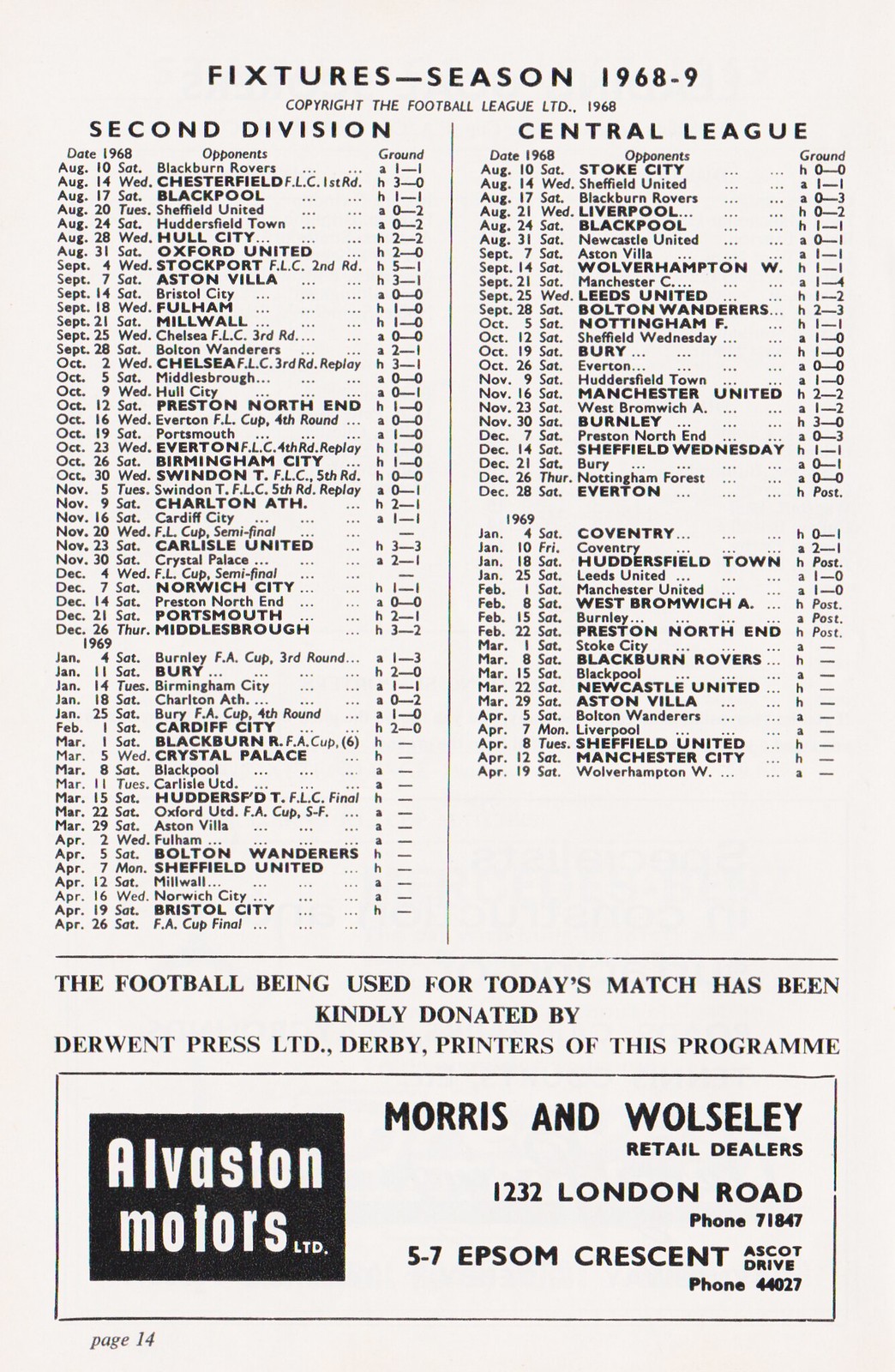The image depicts a page from an old football program, dating back to the 1968/69 season, with a distinctive 1950s-60s font. The title at the top reads "Fixtures Season 1968-9," along with a copyright notice stating "The Football League Ltd 1968." The page is divided into two main columns: "Second Division" on the left and "Central League" on the right.

Each main column is further divided into sub-columns labeled "Date 1968," "Opponents," and "Ground," displaying a list of fixtures and results for the season. The dates range from August 10, 1968, to January 4, 1969, for the Second Division, listing teams like Blackburn Rovers, Chesterfield, Blackpool, Sheffield United, and more. The results indicate whether the matches were home (H) or away (A) and include scores, e.g., "A 1-1" or "H 3-0."

In the Second Division column, notable fixtures include matches against Everton in the FLC 4th Round, Swindon Town in the FLC 5th Round, and a variety of league games. On the other hand, the Central League column lists fixtures against teams like Stoke City, Liverpool, Aston Villa, and Manchester City, also providing details on home and away games with corresponding results.

Below the fixtures, there's an acknowledgment stating, "The football being used for today's match has been kindly donated by Derwent Press Ltd, Derby printers of this program." Additionally, there's an advertisement for Alverstons Motors Ltd, featuring details such as, “Morris & Wolsley Retail Dealers, 1232 London Road, phone 71-847, 5-7 Epsom Crescent Ascot Drive, phone 44027."

Finally, the page number "14" is indicated at the bottom, confirming that this is part of a larger football program booklet from the 1960s.